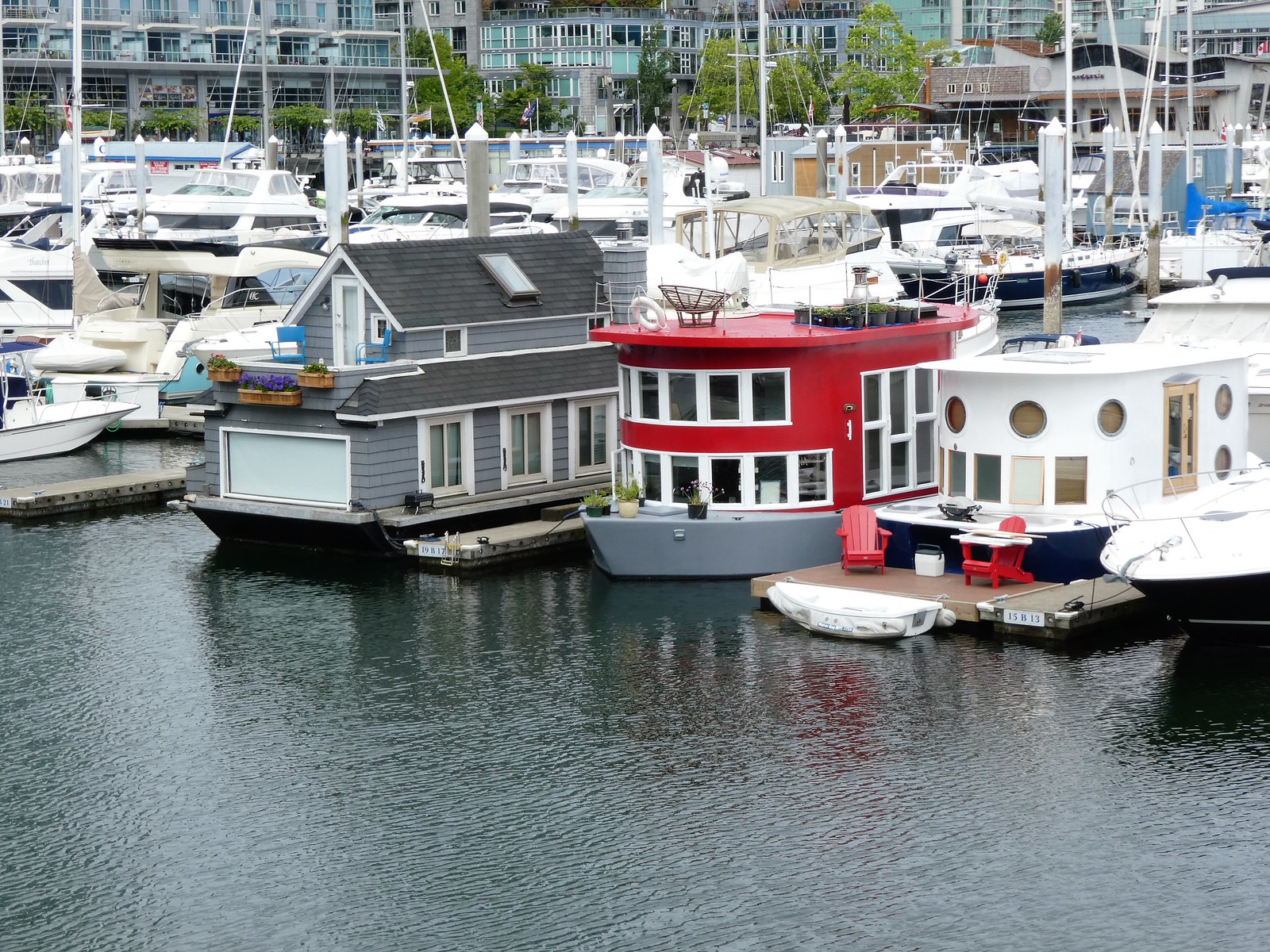This photograph captures a vibrant marina scene with a foreground filled with ocean water and multiple rows of docked boats. The boats are a mix of traditional white yachts and distinctive houseboats. Notably, three prominent houseboats stand out in the foreground: one with a gray house-like structure featuring a garage door-like front and a peaked shingled roof; another with a striking red, multi-story design capped with a deck; and a third white boat boasting round porthole windows and a small patio area with red lawn chairs. The background reveals large, multi-story blue and turquoise buildings, possibly hotels or apartments, with glass windows, partially obscured by a row of green trees. The setting appears upscale, lending an air of luxury to the entire scene.